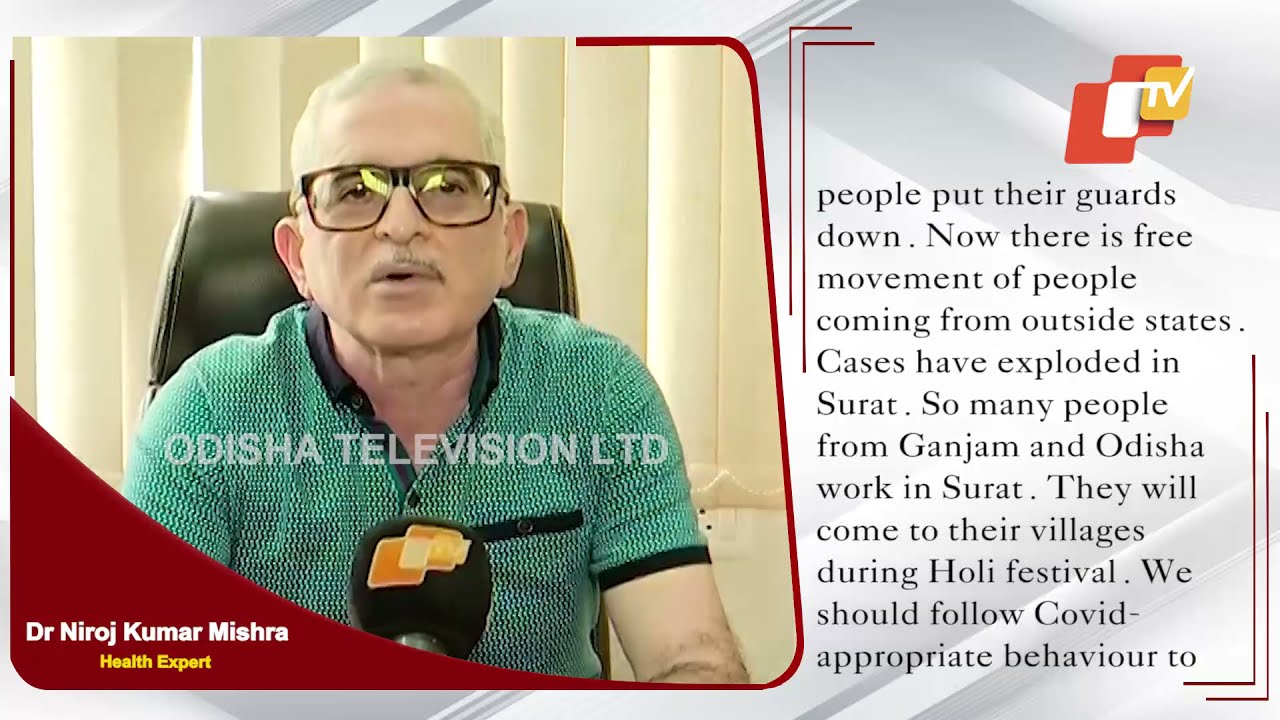The image features an older, light-skinned man with white hair and a thin white mustache, wearing black-rimmed glasses and a green, short-sleeved collared shirt with a black collar, sitting at a desk. He appears to be speaking, evidenced by the microphone in front of him and his mouth slightly open. The background consists of beige vertical blinds. Over his chest, the text "Odisha Television LTD" is displayed in white. In the lower left corner, a red triangle contains his name, "Dr. Neeraj Kumar Mishra," in white text, and below that, "Health Expert" in yellow text. 

On the right side of the image, black text on a white background states: "People put their guards down. Now there is free movement of people coming from outside states. Cases have exploded in Surat. Many people from Ganjam and Odisha work in Surat. They will come to their villages during the Holi Festival. We should follow COVID appropriate behavior." Above this text is an orange logo with the letters "TV." This slide appears to be part of a larger presentation addressing the impact of COVID-19 and the importance of following appropriate safety measures.